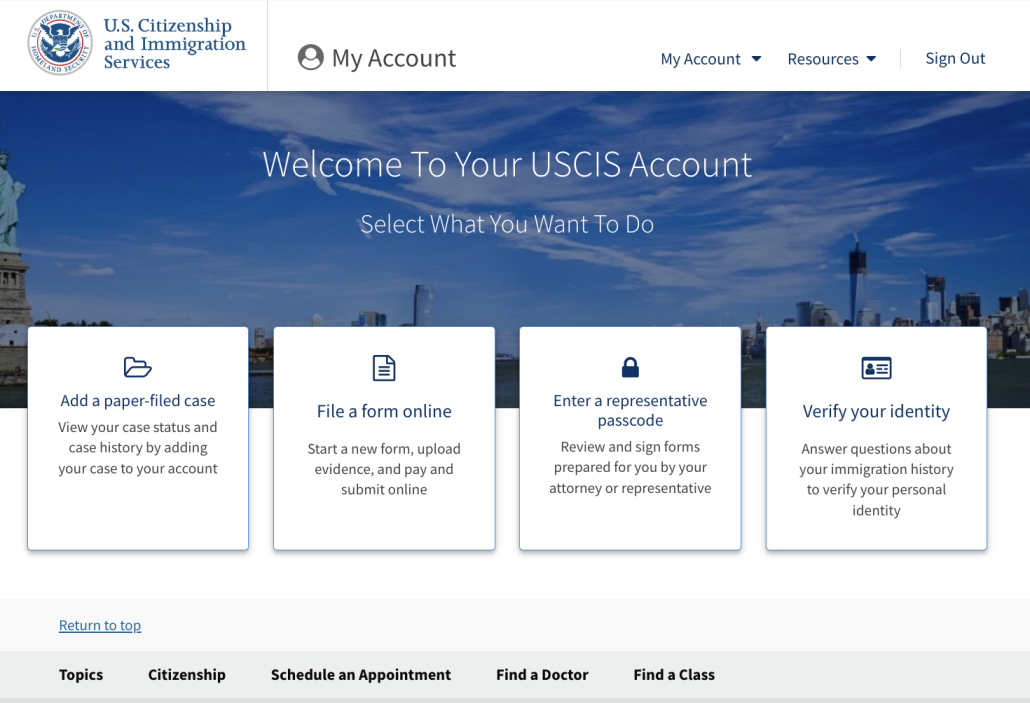The image features a primarily white background at the top.